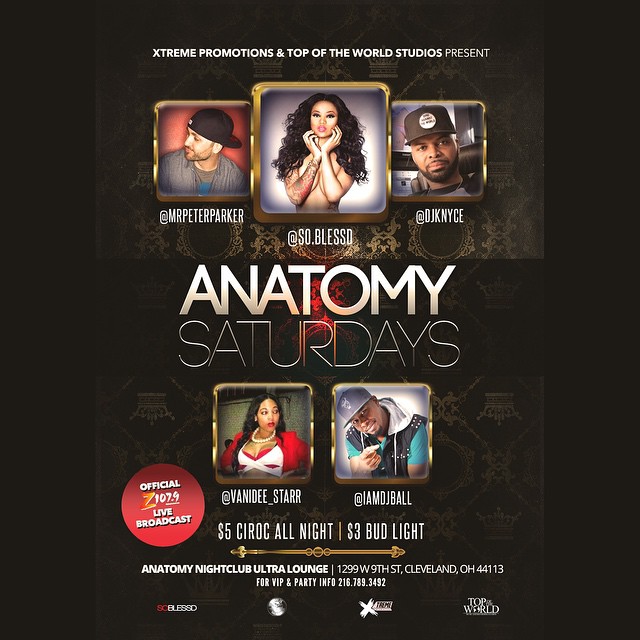The image is a detailed advertisement poster for an event called "Anatomy Saturdays" at Anatomy Nightclub Ultra Lounge, located at 1299 West 9th Street, Cleveland, Ohio, 44113. The background is primarily black, fading to a lighter black with intricate golden symbolism. At the top, it reads, "Extreme Promotions and Top of the World Studios present," followed by five photographs of African American artists with their handles. The first male photo is labeled "@MrPeterParker," the second is a female photo labeled "@so.blessed," the third is a male photo labeled "@DJKnYce," the fourth female photo labeled "@Vanity_Star," and the last male photo labeled "@IAM_DJBall." The text "Anatomy Saturdays" is prominently featured in the center. 

Underneath, it highlights drink specials: "$5 Ciroc All Night," "$3 Bud Light." A round red symbol on the left states, "Official Z107.9 Live Broadcast." Additional information includes "For VIP and party info: 216-789-3492." There are also four logos at the bottom, one for Top of the World, a round Earth-like image, "@SoBlessed," and an X symbol with unreadable text next to it.

The overall design emphasizes a music-related event with live broadcasting, photo images of artists, and special offers, set in an iconic Cleveland nightclub.